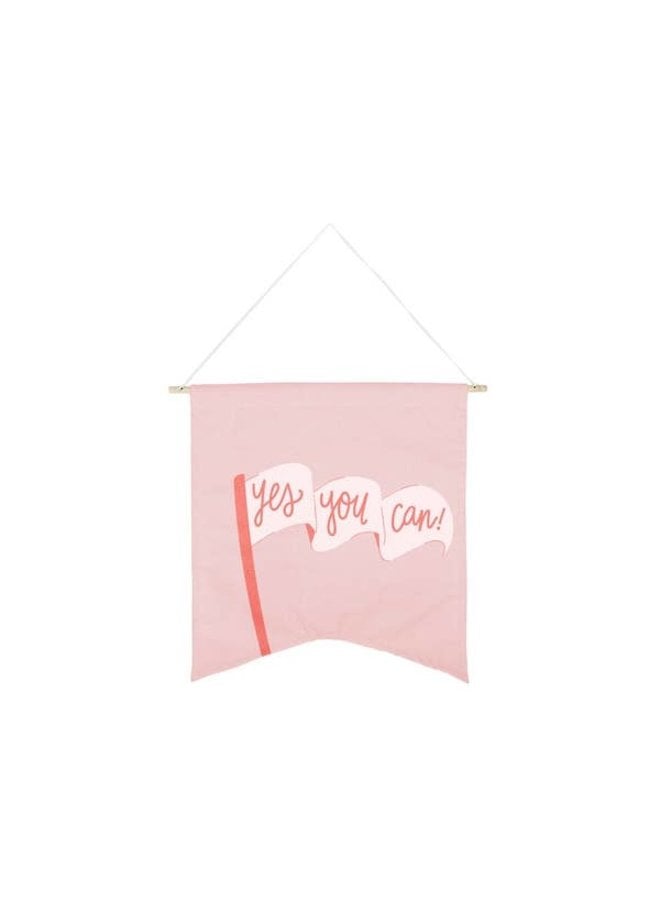The image depicts a pink banner with a salmon-hued vertical line and a feminine cursive message stating "Yes, you can!" in the same salmon color. The design features a flag motif within the banner, where the flag appears to be waving with the motivational text repeated across its folds. The banner exudes a positive and welcoming vibe, reinforced by its soft pink tones. It's hung from a thin rod, likely wooden, by two strings that converge at a central point above, forming a triangle. The background of the image is plain white, emphasizing the banner's simple yet uplifting design.